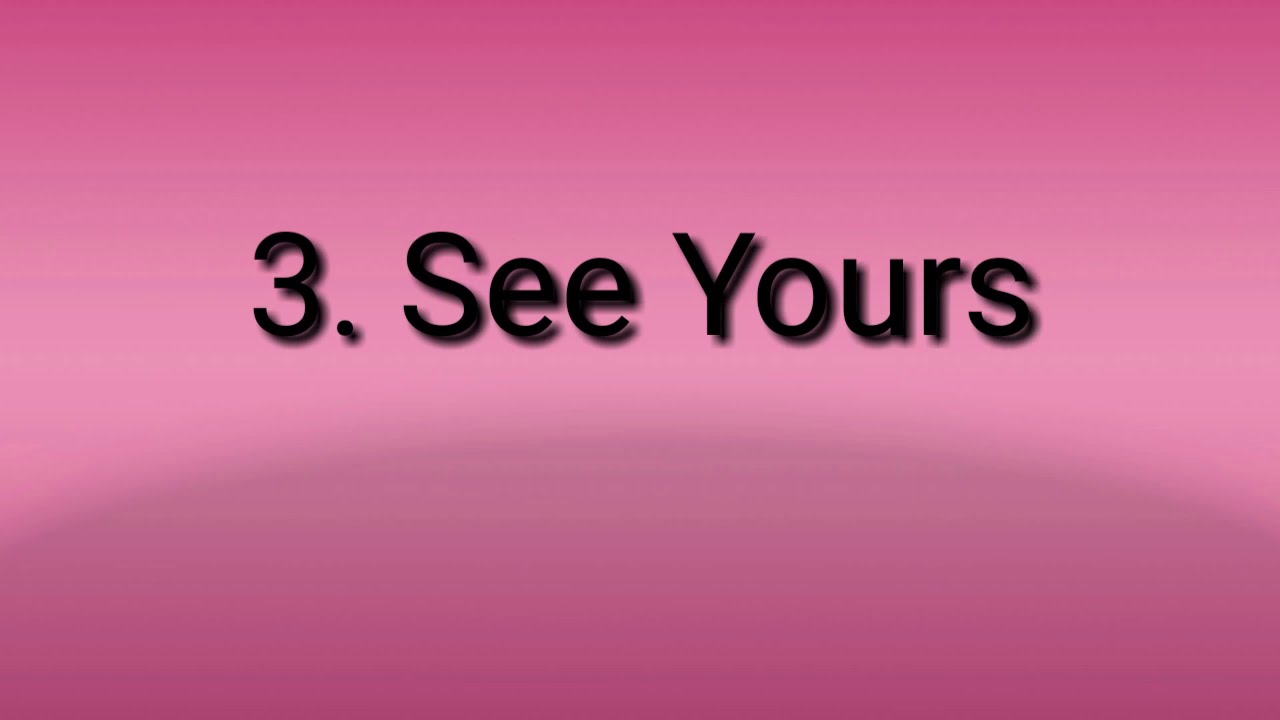This image is a simple and minimalistic design reminiscent of a high-definition television screen, oriented horizontally. The background is a gradient of pink, transitioning from darker shades at the top and bottom to a lighter shade in the middle, with subtle streaks adding texture. In the center of the image, there is white text consisting of the number "3." followed by the words "See Yours," all slightly shadowed to give a three-dimensional effect.